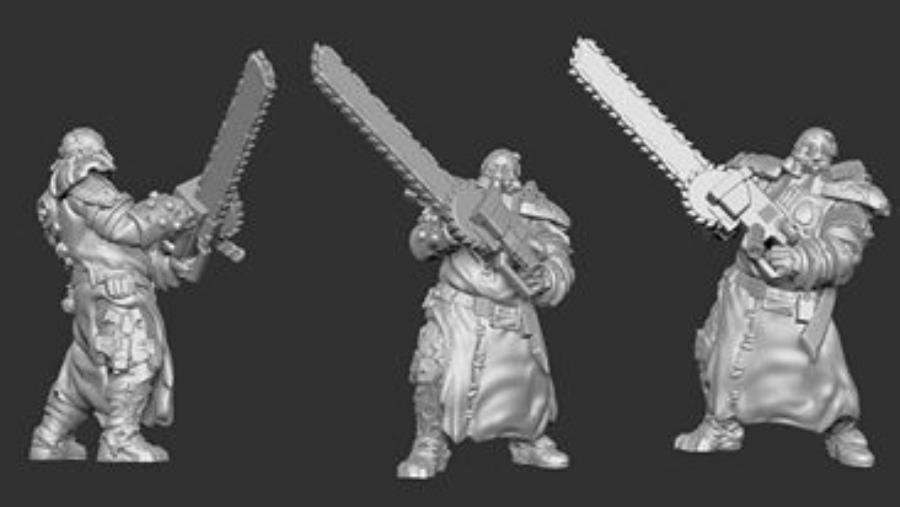The image depicts three silver-gray figurines set against a pitch-black background, giving it a starkly contrasted, almost monochrome appearance. Each figurine, resembling a human or mythical humanoid, holds an oversized chainsaw with wide, jagged teeth, raised menacingly in the air. The figures are garbed in heavy, bulky robes that extend down to their ankles, possibly indicating protection against the chainsaws' imaginary damage. The attire appears lumpy, with potential features like belts, gloves, and shoulder pads, adding to the formidable look. They stand with abnormally wide legs, enhancing their imposing stature, and wear boots. The central figure's right foot pivots forward. The right and middle figurines angle their chainsaws upward to the left, whereas the leftmost figurine angles his chainsaw to the right, facing towards the other two. All heads are bald and are no more than sharp, edged bumps. The entire scene has a cartoon-like essence, with the figures' exaggerated traits and slightly plastic-like texture adding an almost fantastical layer to their menacing pose.